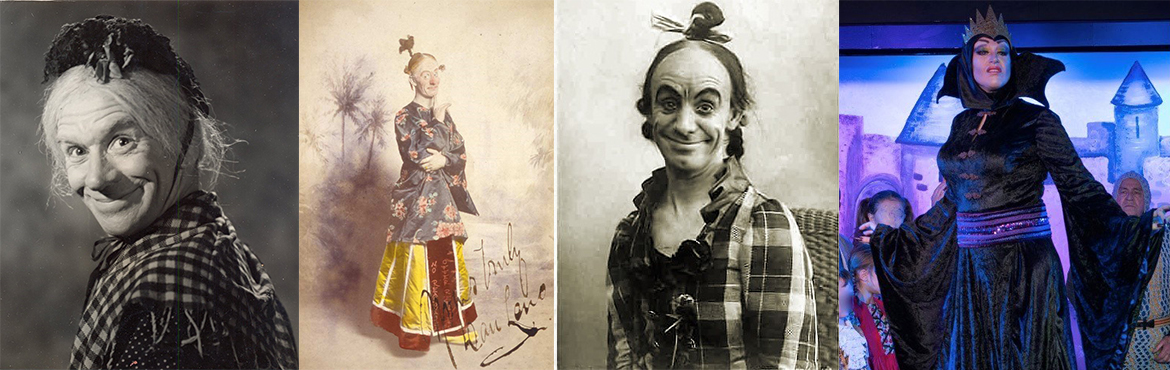This image is a collage of four distinct photographs, each portraying various actors in different character roles, likely from a theatrical production. 

On the far left, the first black-and-white photograph features an older white actor with white hair and wearing black clothing. His expression is a creepy smile as he looks over his shoulder directly at the camera, set against a blurry studio portrait backdrop.

The second photo has a vintage aesthetic, displaying a colorful image of an actor in traditional Asian attire. The background of this photo features a cream-colored wall with tree designs, creating a sophisticated atmosphere. Notably, the foreground includes a discernible signature that reads "Truly, Dan Love."

The third image is another black-and-white photograph, capturing an actor with an unusual jacquard outfit and a peculiar hairstyle. Similar to the first photo, this actor engages with the viewer with a joker-like smile, enhancing the eerie vibe of the image.

The final photo on the right shows a theatrical performance set against a background that includes a castle design. Among the various characters, including children and adults, a central figure stands out—a woman dressed in a black gown and crown, suggesting a witch-like role.

Each photograph contributes to a rich tapestry of characters, varying from intriguingly playful to decidedly unsettling, capturing the multifaceted nature of theatrical performances.